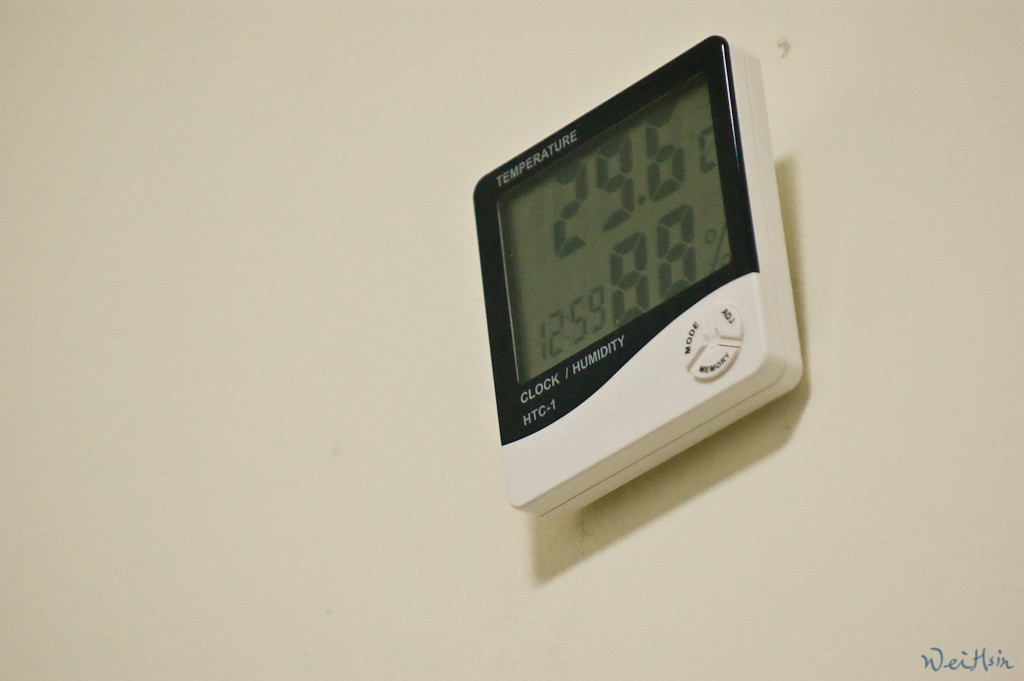This image showcases a digital gauge mounted on a white wall. The device, square in shape and white in color, is encased in a black plastic frame surrounding an LCD screen with black text against a monochrome greenish-gray background. The display prominently shows the temperature as 29.6°C, the time as 12:59, and the humidity level as 88%. Below the display, in large letters, the values are identified with temperature, time, and barometer readings. The device features three slightly raised, white buttons arranged in a pie shape, forming a broken circle. These buttons are labeled in black as MODE, ADJ, and VIEWPORT. The black frame surrounding the screen also has the word "temperature" printed in white. At the bottom of the black frame, the model identification "CLOCK / HUMIDITY HTC-1" is visible.